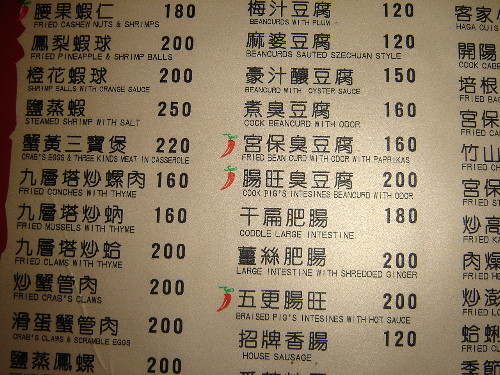The image depicts a Japanese food menu featuring an elegant beige background. The menu is densely populated with black text, which consists of both Japanese characters and corresponding prices. The layout is structured to guide the diner through an array of culinary options. Each item is meticulously listed, ensuring clear readability and an authentic representation of traditional Japanese cuisine. The overall design emphasizes simplicity and functionality, making it easy for patrons to navigate through various food choices.